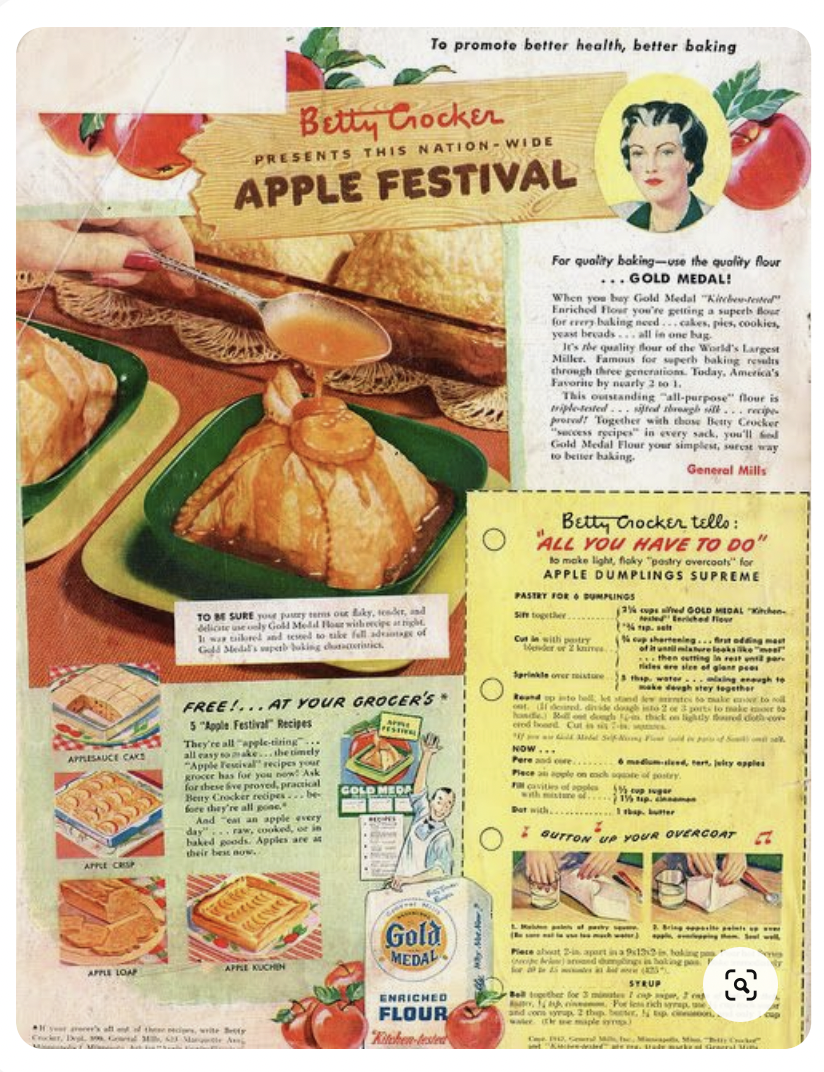This image appears to be a page from a cookbook or magazine, likely an advertisement for Betty Crocker's nationwide Apple Festival. The background features a mix of white and yellow, with the prominent Betty Crocker logo at the top. Below the logo, it reads, "Betty Crocker presents this nationwide Apple Festival" in bold black text on a wooden signboard design. The upper section discusses promoting better health and baking, with accompanying text by General Mills about their Gold Medal flour. There's an illustration of Betty Crocker, depicted with black hair, a blue and green shirt, red lips, and a yellow background, flanked by red apples with green leaves. 

To the left, there's an image of a person spooning what appears to be an apple glaze or caramel drizzle over a white dessert, possibly apple dumplings, on a green plate. On the right, a text box promotes using Gold Medal flour for quality baking, with additional bold black text highlighting various apple-related recipes available for free at grocers: applesauce cake, apple crisp, apple loaf, apple kuchen, and apple dumplings supreme. 

A dotted line with three black circles creates a border around another section that emphasizes baking tips from Betty Crocker, alongside an illustration of a man in a white apron, black bow tie, and blue shirt, presenting a package of Gold Medal flour with noted features such as "enriched" and "kitchen tested." The lower part includes vibrant details of red apples and music notes, enhancing the festive theme of the Apple Festival.